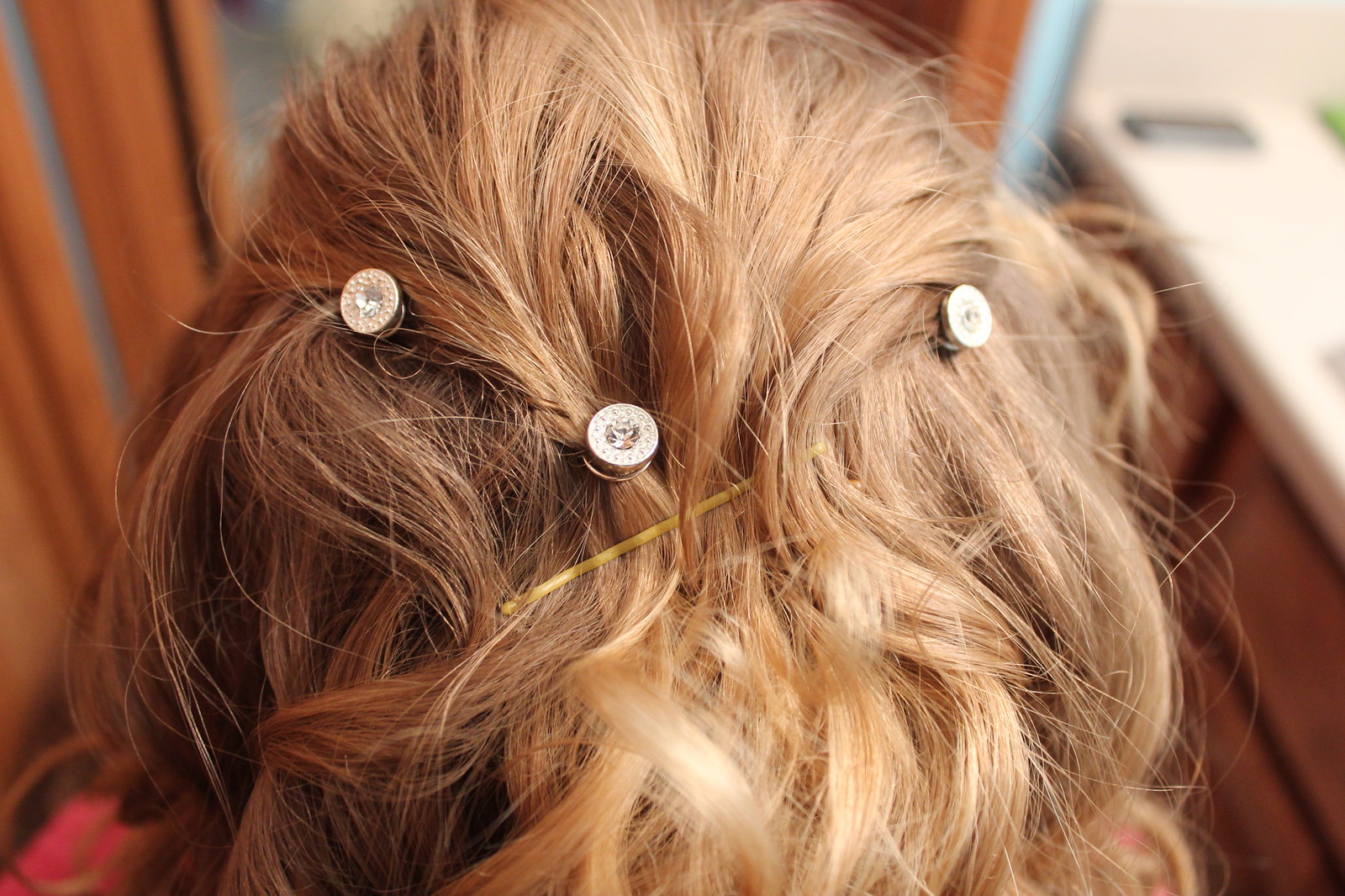The image captures a close-up of the back of a young girl's head, showcasing her strawberry blonde, gently wavy hair. Her hair is intricately styled with numerous clips and decorative elements. On her left side, she has a silver round clip placed towards the upper section of her hair, and a matching clip a few inches below it. Underneath these, a thin gold bobby pin subtly blends into her hair. Interspersed among these clips are three small, rounded hair jewels, pale gold in color, featuring cubic zirconia-like stones in their centers, adding a touch of sparkle. On the right side, another clip secures her hair. The background is slightly out-of-focus, revealing hints of an indoor setting with orange walls, a countertop to the left, and bright white lighting illuminating her hair.